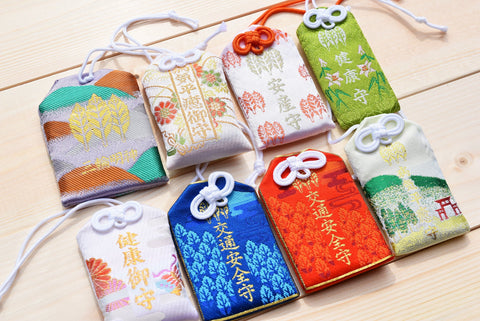The image depicts eight small, handmade Japanese amamori, each uniquely designed and displayed on a light brown wooden surface, possibly a porch or table. The amamori vary in color, featuring shades of teal, brown, white, green, blue, gold, red, and there are prominent dark blue and red ones. Each has intricate designs and symbols, including kanji characters. They are arranged in two rows of four, and all have bows or tied knots at the top, likely for hanging or securing, and resemble gift bags or tags. Notable designs include the leftmost amamori on the top row, which is dark blue with aqua and brown hill-like structures and three golden leaves in the center. Some also incorporate Chinese symbols as part of their decoration, indicating a festive or cultural significance.